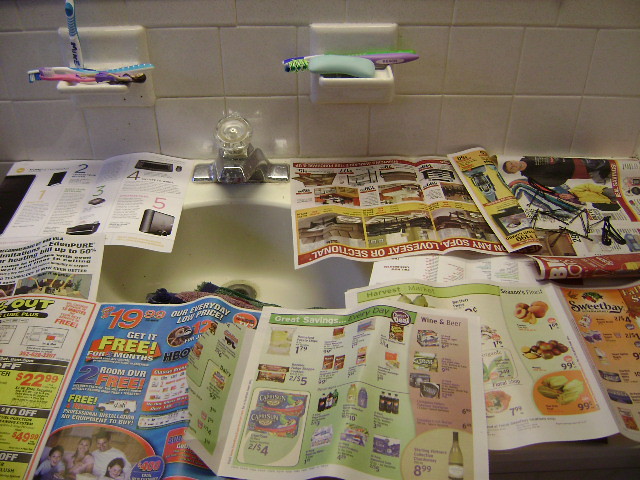In this detailed image, the focal point is a bathroom sink scene. Displayed prominently on the sink are multiple items of everyday use. To the left, there is a holder, presumably made of tile, containing about four or five toothbrushes in various colors—pink, purple, blue, and white. A horizontal brush lies behind a light teal or blue bar of solid hand soap which sits in a soap holder. The surrounding area above the sink features whitish sporting tiles, with at least three rows visible on the back wall, although the top row is only partially captured in the frame. 

Scattered on top of the sink are different newspaper advertisements. Inside the white sink, slightly discolored due to lighting or slight dirt, there appears to be some cloth or another ambiguous object. The chrome faucet stands out with its clear plastic handle. This intricately detailed capture provides a glimpse of an everyday bathroom setting, complete with all its nuances and details.